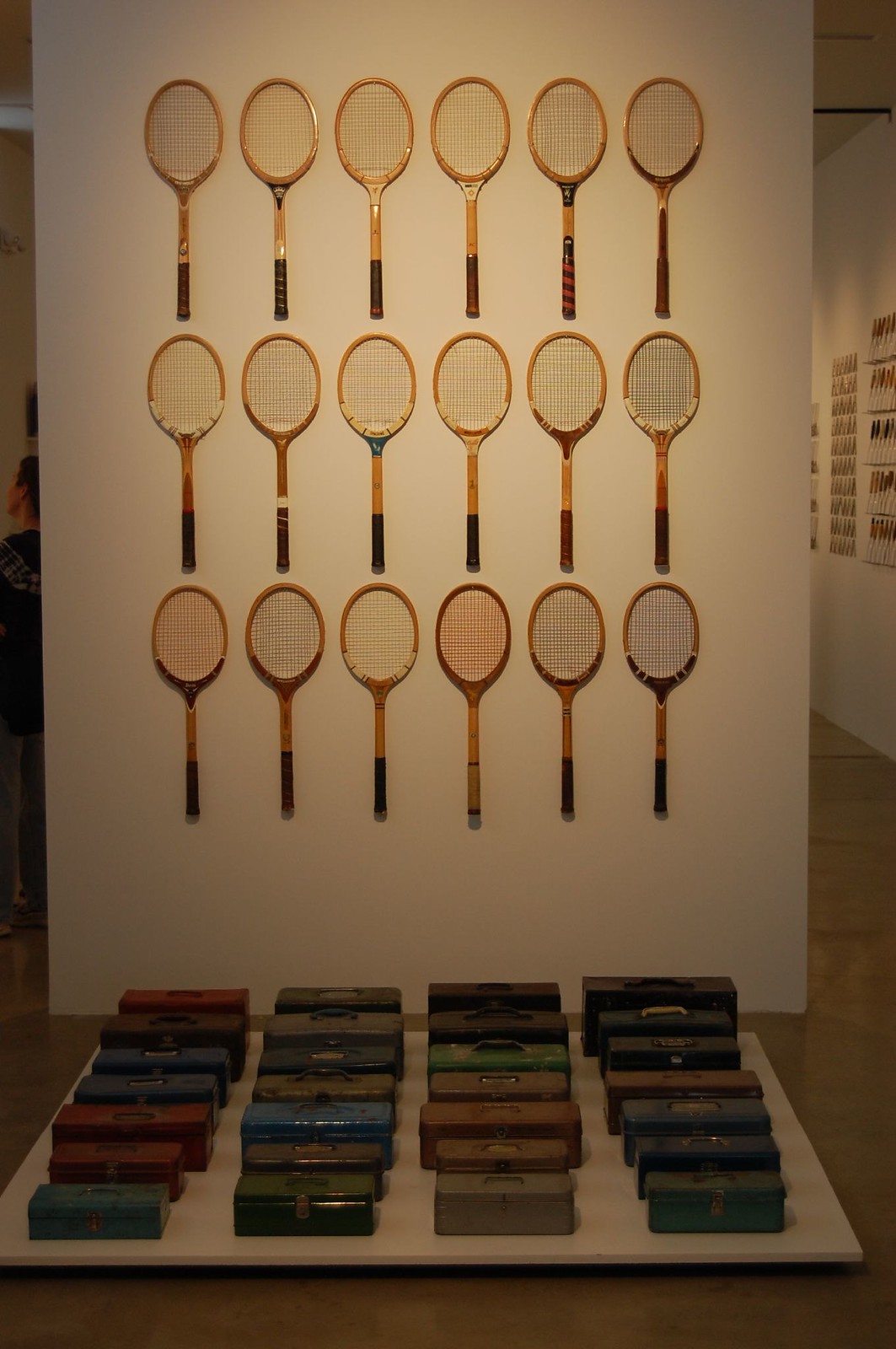The image portrays a vertically oriented photograph taken indoors, possibly in a museum or gallery, showcasing a meticulously arranged art display. The scene, bathed in a warm tungsten light that imparts a reddish-yellow tint, features 18 wooden tennis rackets mounted symmetrically on a white wall. The rackets are organized into three rows of six, with each racket's oval portion pointed upward and the wooden handle downward. Below them, placed on a separate white platform, are 28 small, rusted metal toolboxes. These boxes are organized into seven rows of four and exhibit a variety of colors, including green, blue, orange, brown, and red, contributing to the overall aesthetic of the display. The setup creates a compelling visual symmetry, enhanced by the texture of the rackets' netting and the multicolored, weathered toolboxes. The wooden gallery floor and surrounding walls with more symmetrically arranged pieces complete the setting, underscoring the precision and artistic intention of the exhibit.